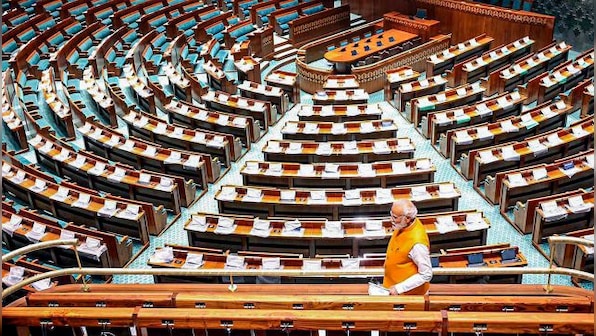The image depicts an expansive lecture hall or governmental assembly room featuring multiple tiers of seating that surround a central area. The individual in the foreground, who resembles Indian Prime Minister Mahindra Modi, stands on an elevated balcony or higher level. He is dressed in a white long-sleeved shirt paired with an orange puffer vest, with distinctive white hair, a gray beard, and glasses. The hall's seating arrangement is intricate, with rows of chairs that point towards the middle of the room, where a prominent wooden table is set up. This table is flanked by ten chairs, five on either side, and is equipped with computer monitors. Additionally, the scene includes a podium and a stage behind the table, and all of the seats in the hall are depicted as empty. The auditorium is adorned with seats of two different colors, possibly orange and green, adding a vibrant touch to the structured setting.